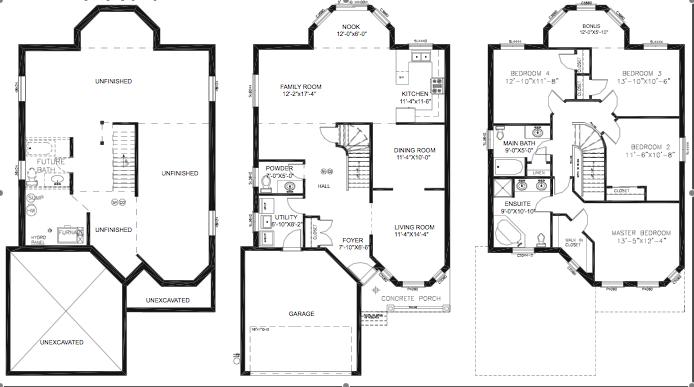**Caption:**

A detailed architectural blueprint of a proposed three-storey building rendered in black lines on a white background. The structure comprises a long rectangular main body, with an additional square section designated as the garage located at the bottom left-hand corner. Notably, a bay window is notched out at the top of the rectangular outline. 

The first level, marked as "unfinished" in multiple areas, features lightly sketched dotted lines indicating the potential placement for a future bathroom and includes a centrally located stairwell.

Moving up to the second, or middle level, the floor plan includes various living spaces such as a nook, family room, kitchen, powder room, utility room, foyer, dining hall, and living room. A distinct feature of this level is a slightly curved central stairwell, and a concrete porch extends out from the living room area.

The topmost level showcases the private living quarters with designated spaces for a bonus area, four bedrooms (including a master bedroom with an ensuite), and a main bathroom. The blueprint notably leaves the areas corresponding to the garage and concrete porch below unmarked, indicating no additional construction in these sections at this level.